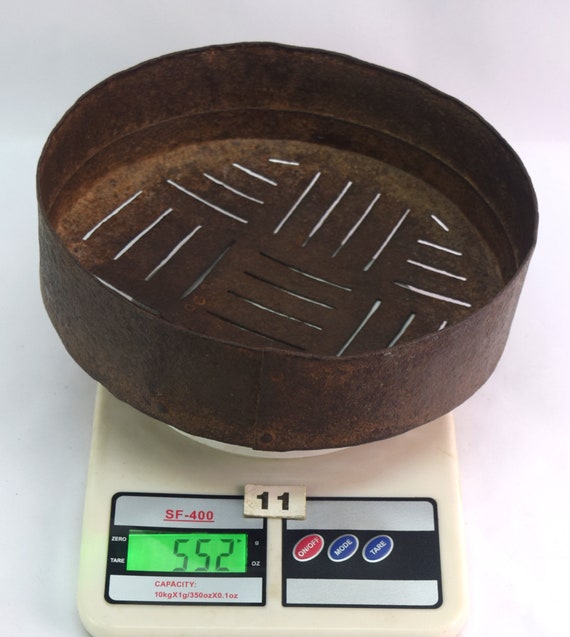This detailed image captures a vertical rectangular photograph of a white digital kitchen scale set against a white or gray backdrop. Centered on the scale is a small, round, metal container with noticeable rust and a brownish hue, indicative of frequent use and possible water exposure. The container features a series of crisscrossing lines or slits at its base, resembling a grill pan that might leave grill marks.

The digital scale prominently displays an LED screen reading "552," presumably indicating the weight in grams. Above this display, the label "SF-400" can be seen in red, while below it, specifications are listed as "Capacity 10kg x 1g / 350oz x 0.1oz." Additionally, there is a white rectangular label with the number "11" in black situated on the front of the scale.

To the right of the LED screen, three buttons are visible: a red "On/Off" button, a blue "Mode" button, and a blue "Tare" button. The overall scene presents a simple yet detailed snapshot of a frequently used kitchen scale with a weathered metal container poised on top.